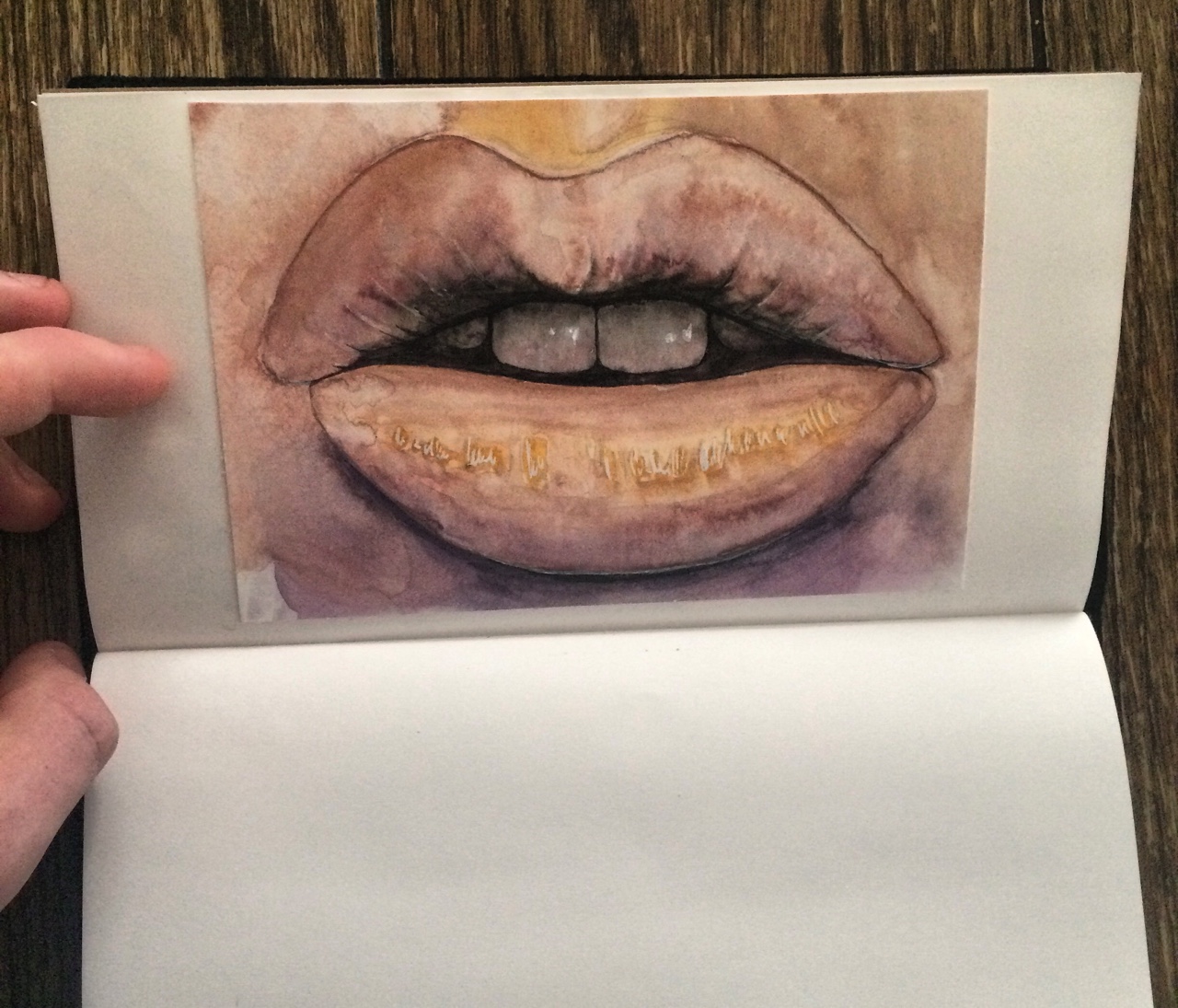In the image, an open notebook is positioned sideways on a dark brown table, with one page standing upright and the other lying flat. A left hand with four fingers is visible on the left side of the notebook. The notebook itself has a white background, and the upright page features a detailed drawing of a pair of lips with a couple of teeth visible on the top row. The artwork is accentuated with cursive white lettering outlined in gold. The lips are set against a background shaded in brown, purple, and a hint of yellow at the very top.